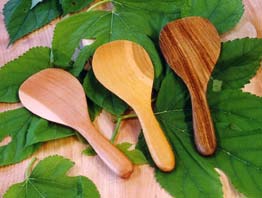The image displays three differently colored wooden spoons arranged from right to left atop a spread of vibrant green leaves on a pink surface, likely a table. The spoons exhibit various shades and textures: the spoon on the right is a dark brown resembling walnut, the middle one is a yellow-brown, possibly oak, and the leftmost spoon is a pale brown, almost pinkish hue. Each spoon has a thin handle that broadens into a paddle-like shape, indicative of basting spoons rather than circular spoons or spatulas. The scattered leaves beneath the spoons conform to their shapes, enhancing their soft, leafy textures. The entire arrangement rests on what appears to be a wooden table painted a striking pink, adding a vivid backdrop to the scene.